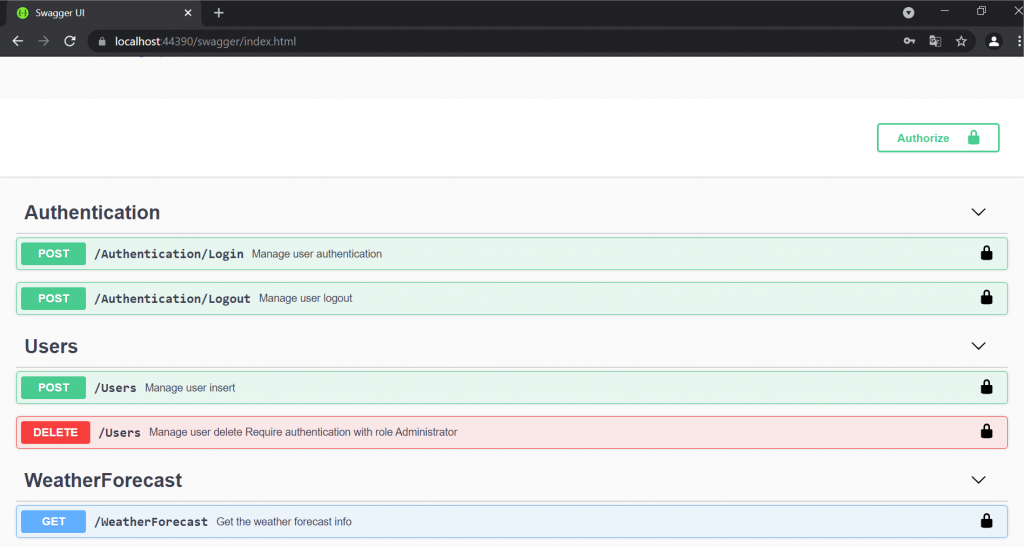This image captures a web browser interface with a single tab open for Swagger UI, showcasing an organized layout for API documentation. The browser's display window predominantly features a black bar at the top, while the page itself has a clean white background. The address bar displays the URL "localhost:44390/swagger/index.html." To the left of this address bar, there are back and refresh buttons. Next to the open Swagger UI tab, there's an icon for adding new tabs, represented by a plus sign.

The Swagger UI is divided into three main sections, each clearly delineated and containing various controls for API interactions:

1. **Authentication**: This section contains two rows, both marked by green "POST" buttons, indicating endpoints for creating or managing authentication tokens.
   
2. **Users**: This section also has two rows; the first with a green "POST" button for adding users and the second with a red "DELETE" button for removing users.

3. **WeatherForecast**: Written as one word, this section has a single row colored blue with a matching blue "GET" button for fetching weather forecast data.

Additionally, at the top right corner of the browser, there is an "Authorize" button featuring a green lock icon, which likely serves to manage API access permissions. Each row within the three sections also includes a small lock icon on the far right, presumably for securing the respective actions. 

Overall, the image provides a detailed view of an API management and testing interface, highlighting the functional and user-friendly design of Swagger UI for developers.